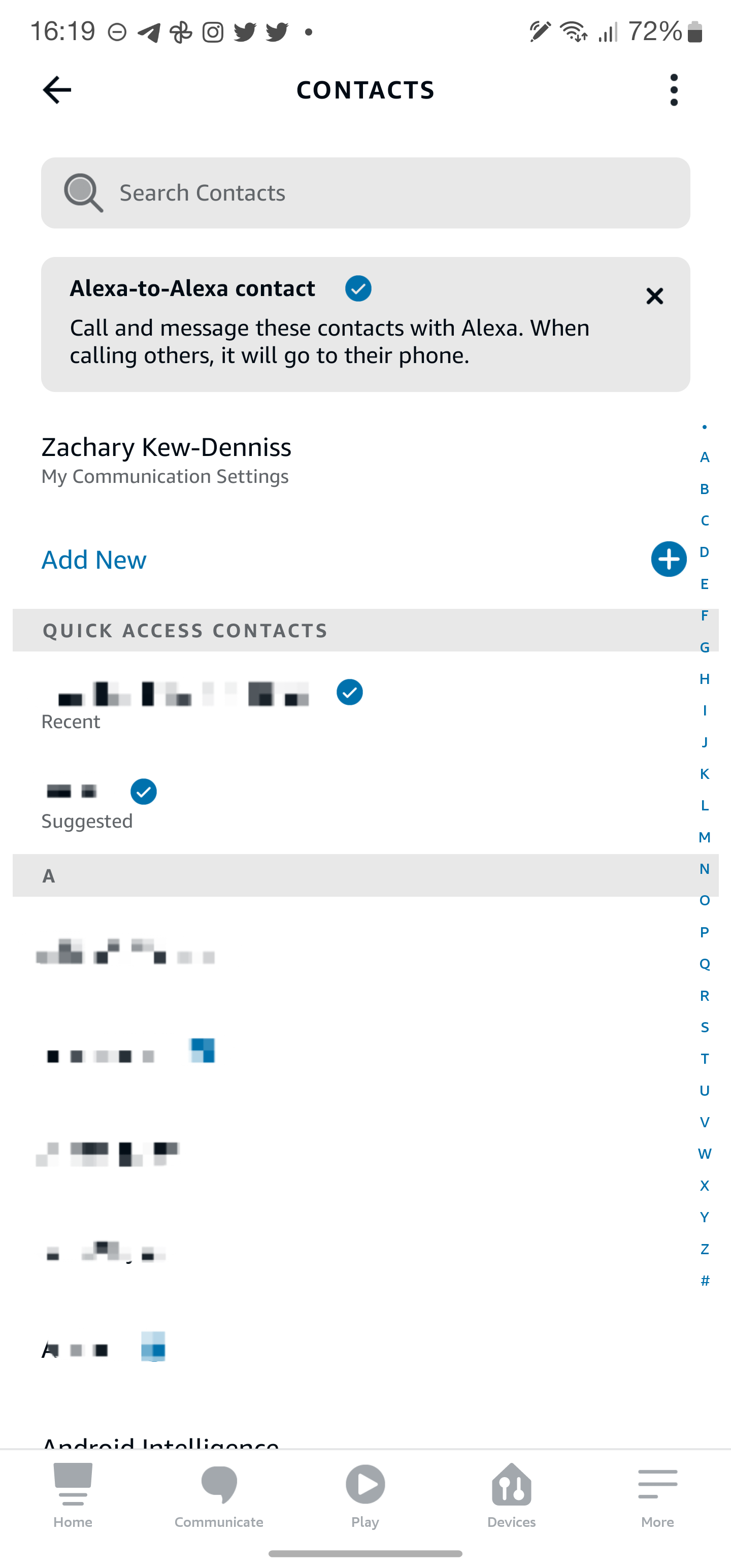The image depicts a contact management screen on a smartphone, showing several key features and interface elements. At the top of the screen, there are various status icons including the time (16:19), a Pinterest logo, a pinwheel icon, two Twitter logos, Wi-Fi signal strength, a pen icon, cellular signal bars, and a battery icon showing 70% charge.

Immediately below these icons is a search bar labeled "Search Contacts". Under this, there's a section for "Alexa to Alexa Contact," with a note indicating that you can call and message your contacts via Alexa. The screen also mentions that calls made to others will be directed to their phone.

The contact list starts with "Zachary Q. Dennis," accompanied by a subsection labeled "My Communication Settings." A vertical A-to-Z index appears in blue on the right side of the screen for easy navigation through contacts.

Several features are noted but pixelated out, including "Add New," "Quick Access," and what seems like a batch of check-marked items under "Suggestions." The 'A' section shows five pixelated results, partially cut off by a scroll bar.

At the bottom of the screen, an Android navigation menu includes the following icons: 
- "Home" represented by a house icon.
- "Communicate" depicted by a speech bubble.
- "Play" indicated by a circled arrow.
- "Devices" shown as lines with dots inside a home icon.
- "More," although not detailed in the description.

The image showcases the intricate layout of a contact management interface on an Android smartphone, complete with interactive elements and organizational features.